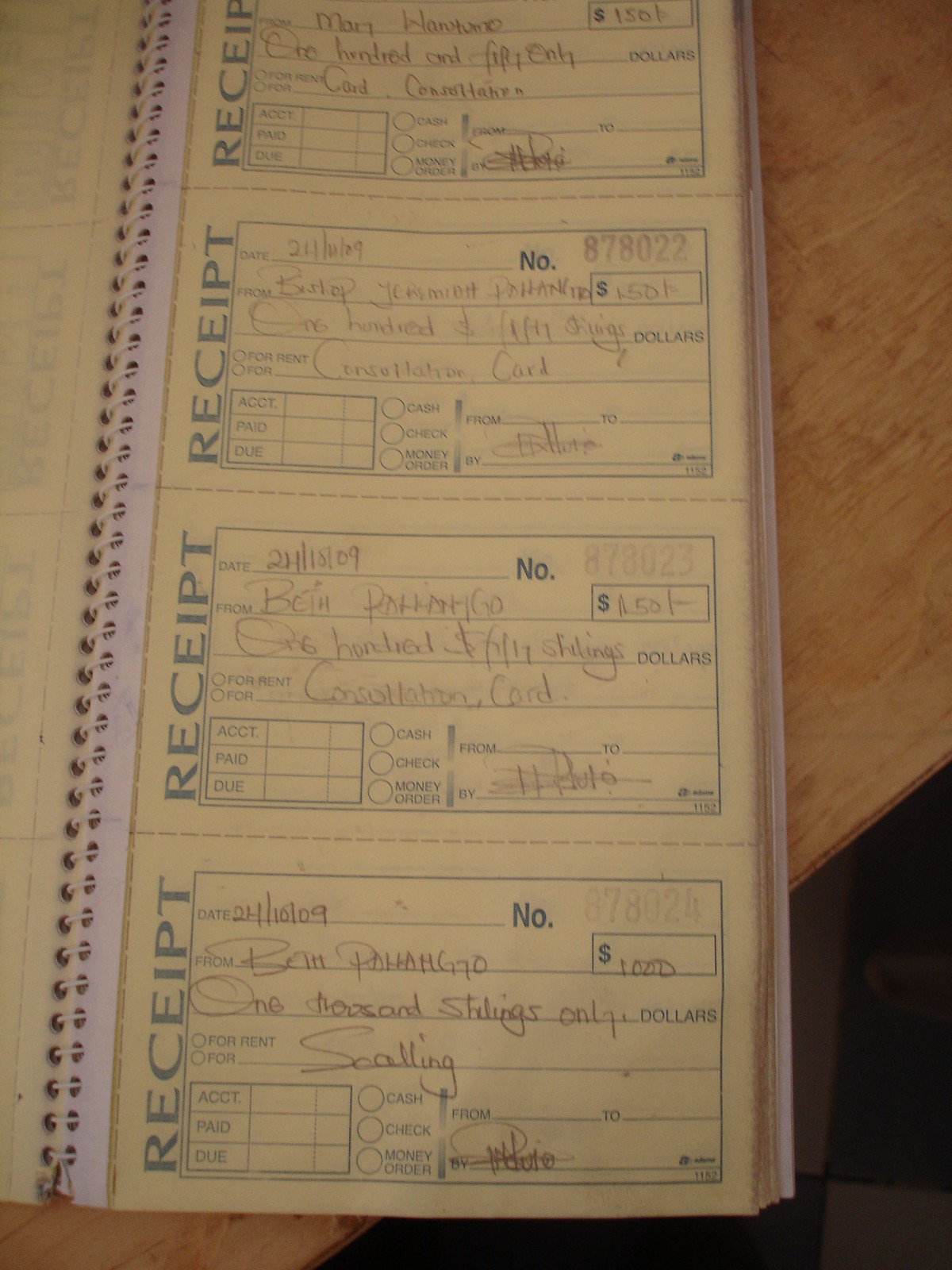The image captures a partial view of a long, slender spiral-bound receipt book with a rectangular shape. This old-fashioned, journal-like receipt book features a white wire binding running along its length, allowing easy tear-out of the perforated yellow receipt pages. Each page contains four receipts, all of which are completely filled in with detailed entries. The receipts include numbered and dated transactions written by hand, such as one dated 10-24-2009, indicating an amount of $1,000 to a person named Beth. The receipts have the word "receipt" printed vertically in blue along the sides. The book is placed at an angle on a thin, light-colored wooden table, with the bottom right edge hanging off, revealing a black and white checkered floor and a dog's foot in the bottom right corner. The entire scene is slightly blurry, but the details of the handwritten receipts are still discernible.